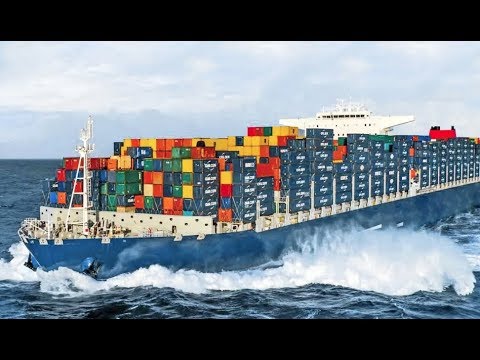A massive blue container ship sails diagonally through the choppy dark slate sea, with its bow crashing into waves, creating a visible spray on the right side. The sky above is a pale blue with grey clouds stretching towards the horizon, interspersed with some white fluffy clouds directly above the vessel. The ship, towering with a white bridge and tall structure at its front, is fully loaded with shipping containers, stacked like a colorful array of Lego blocks. Predominantly blue containers line most of the visible side, with scattered red, yellow, green, and orange containers adding bursts of color. Despite the rough sea, the ship appears to be navigating effortlessly, making its way to an unknown destination.